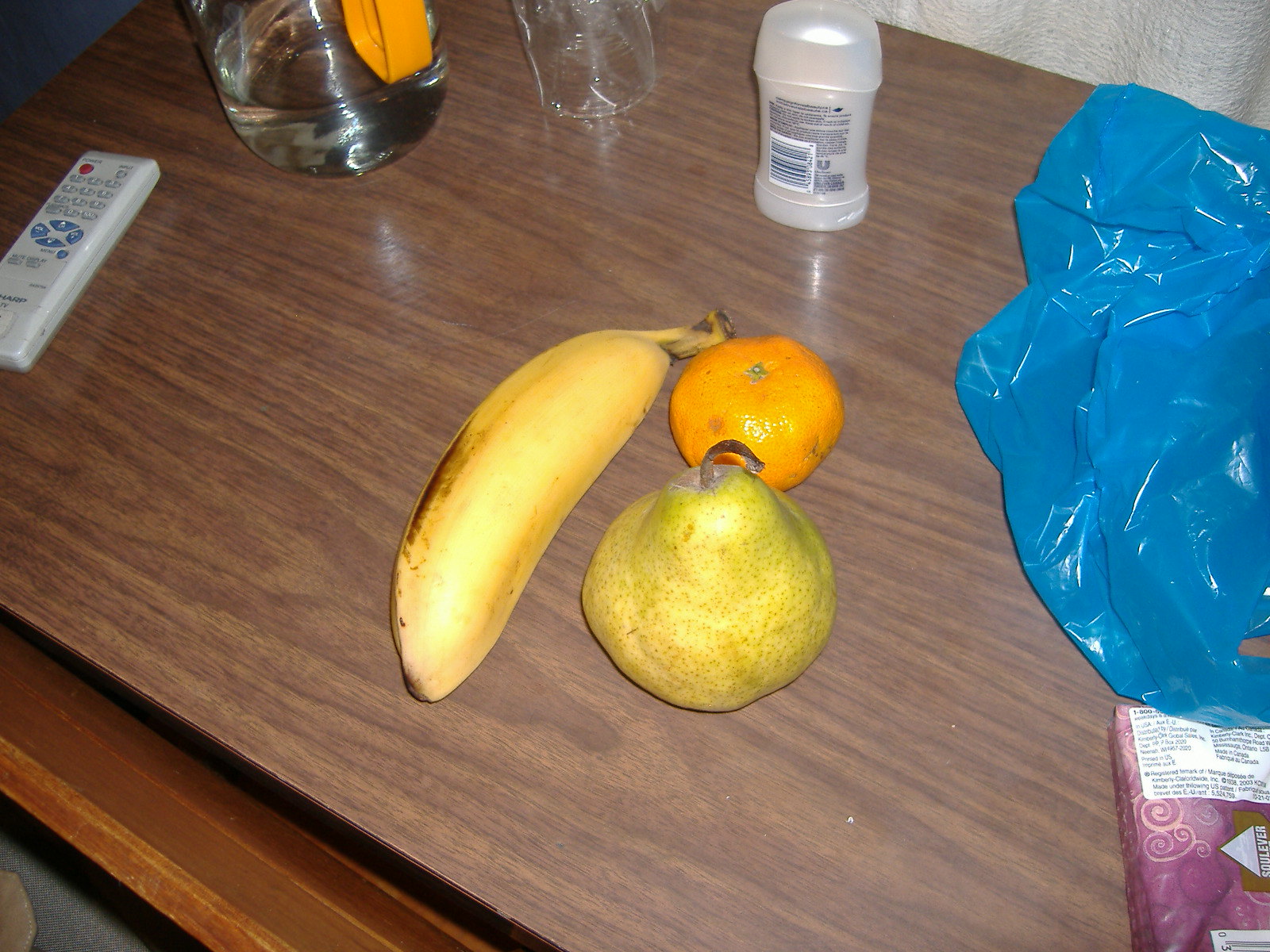The image depicts a hospital bedside table with a variety of items neatly arranged on its surface. The table itself is reminiscent of those often found in hospital rooms, designed to slide over a patient's bed for easy accessibility. Adjacent to the table is a curtain, further suggesting a hospital setting.

On the left side of the table, there is a remote control positioned beside a bottle or glass of water. Nearby, a clear plastic container holds an unidentified item. Also present is a deodorant container, which appears to be either Dove or Secret brand.

Closer to the viewer, a banana, a clementine, and a pear are arranged together. The banana is notably straighter and stouter than usual, with some browning on its side, though still seemingly edible. The clementine and pear also appear to be in a consumable state.

To the right, there is a small pack of tissues, the kind typically carried in a purse or backpack. Above these tissues sits a blue, opaque plastic bag. All items are organized on the tray, contributing to the overall impression of a hospital environment.